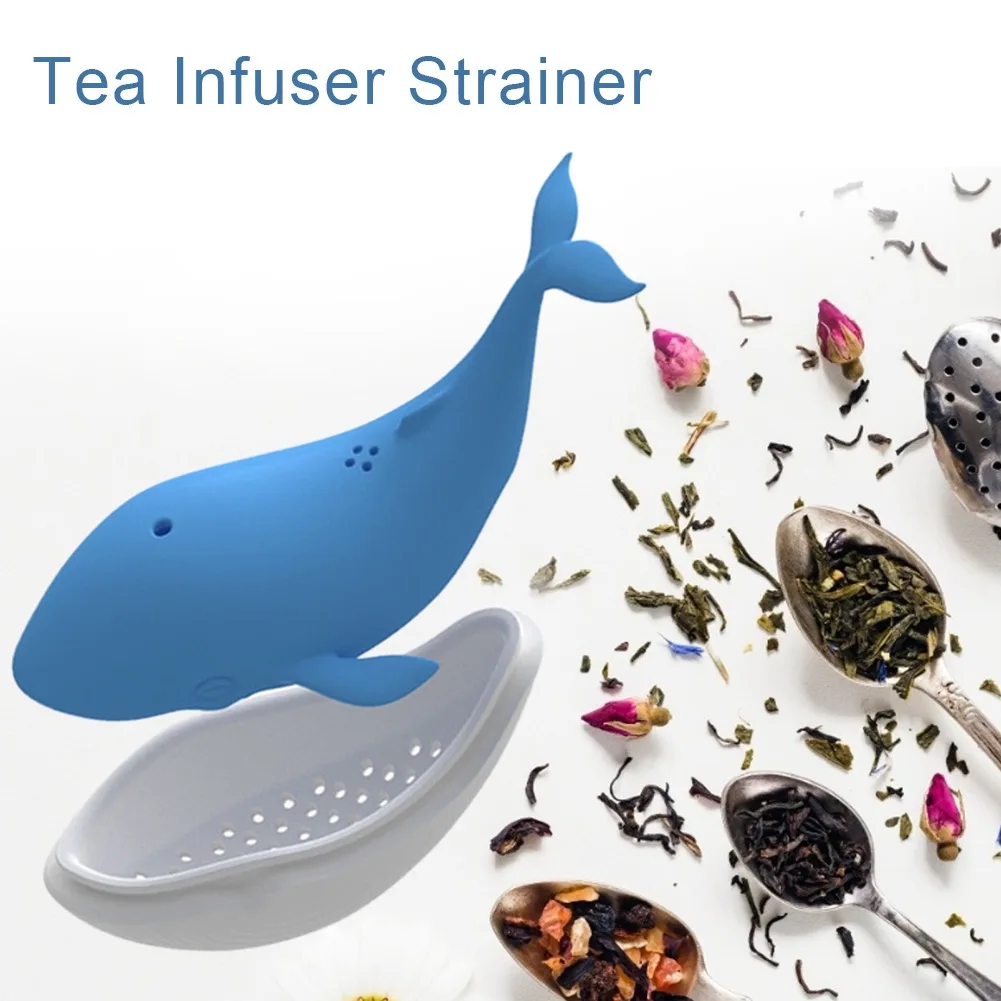This image features an advertisement for a tea infuser strainer, prominently labeled in blue text at the top left corner against a white background. The central product is designed to resemble a blue whale, complete with a detailed plastic exterior and a white underbelly that functions as the strainer. The whale's design includes five small holes: one where a blowhole would be, and four arranged in a diamond shape towards the tail fin. The detachable white base of the infuser, representative of the whale's belly, is oval-shaped and peppered with multiple perforations for effective straining. To the right of this main image, the white background showcases an assortment of spoons, each filled with various dried herbs, leaves, and flower buds. These spoons, alongside a metal tea strainer in the top right corner, further emphasize the tea preparation theme. The scattered herbs and leaves on the backdrop add a natural, aromatic element to the overall composition.